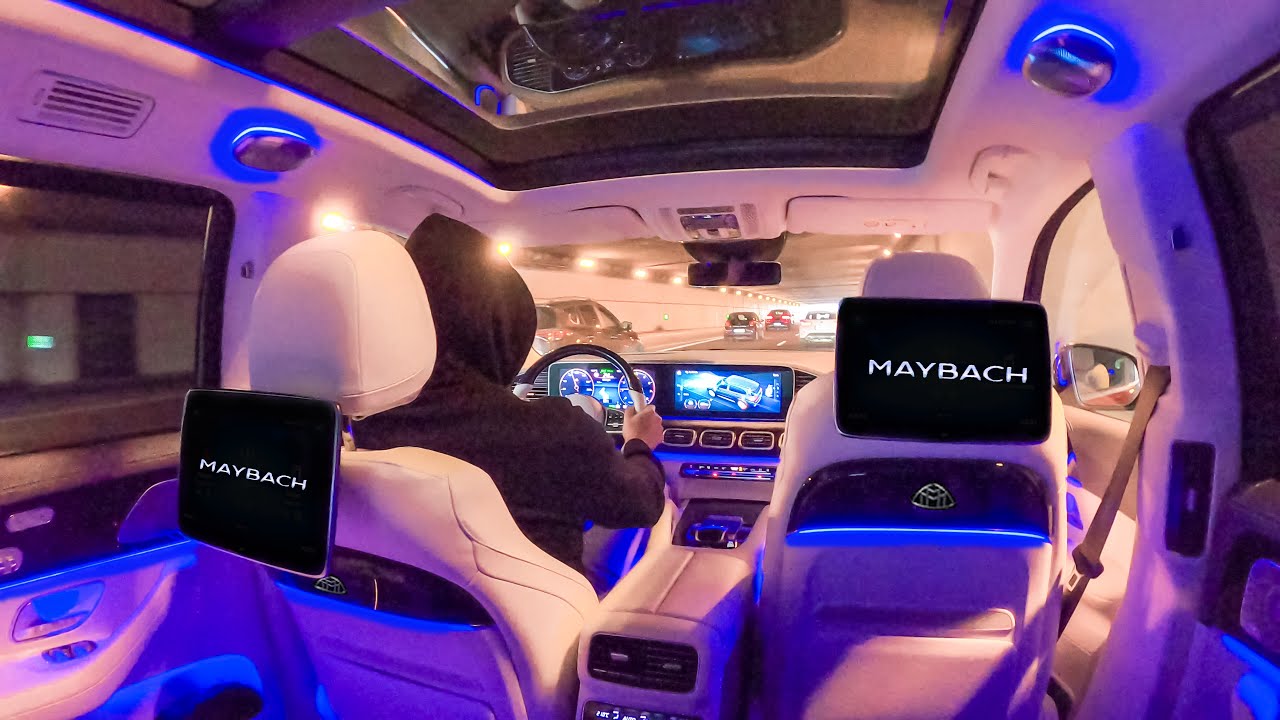The image depicts a highly advanced and luxurious Maybach vehicle from the perspective of the back seat, rendered in a photorealistic CGI or AI-generated style. The interior is bathed in shadows of neon purple and cobalt blue light, enhancing the opulent atmosphere. A driver, dressed in a black hoodie with their hands on the wheel, is seen navigating through a tunnel, with three other cars visible ahead through the front windshield. The spacious, light-colored (tan) interior features a large moonroof and an extensive array of technology, including prominent video screens on the back of both the driver's and passenger's seats, each displaying the Maybach logo. The central console hosts another sizable screen showing a live feed of an approaching van. Blue LED light trims accentuate the seats and doors, contributing to the futuristic ambiance of the vehicle.